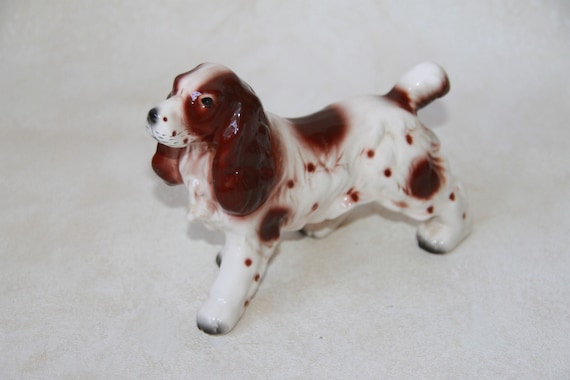This is a highly detailed full-color photograph of a small dog figurine, likely made of ceramic or porcelain, staged and taken indoors under artificial lighting. The image showcases a side view of the figurine, which appears to be a Cocker Spaniel or Beagle with distinctive features. The figurine is positioned on a light gray background, and the photo is horizontally rectangular without any discernible border. 

The dog has long, floppy ears that are primarily brown, a white muzzle with a white streak running across its head, and a black nose. The body of the figurine is predominantly white, adorned with several brown patches, including a brown dot in the center of its back, another on the thigh, and one near the front armpit area. Additionally, smaller black dots speckle the lower parts of its legs. The figurine's tail is short, and its stance includes a slightly extended front paw and a back paw positioned farther back. A shine from the artificial light highlights the head and tail areas, adding a touch of realism. Shadows cast by the figurine onto the countertop enhance the three-dimensional effect.